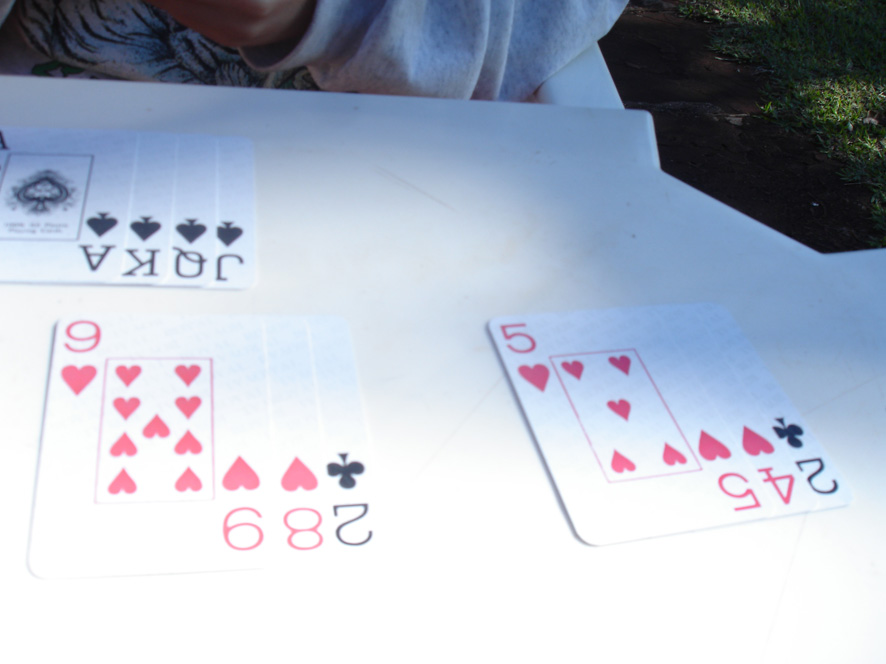The image captures a set of playing cards arranged on a white surface. The cards, primarily white with detailed suits and numbers, display a variety of designs. Starting from the right, there is the 5 of Hearts followed by the 4 of Hearts, then the 2 of Clubs in black. Further left, there's another 2 of Clubs, the 8 of Hearts, and the 9 of Hearts, both in red. Notably, one of the 9 of Hearts cards also shows multiple hearts, numbering 2, 4, 6, 8, and 9 hearts inside the rectangle, along with one beneath the numerical value. 

Above these cards, a series of cards showing the letter J, Q, K, and A with black spades can be seen. They are set against what appears to be a white table surface. In the background, to the top right, there is a well-maintained green grass lawn and a brown pavement. Additionally, on the left side of the image, part of a cream-white cloth is visible along with a white hand emerging into the frame.